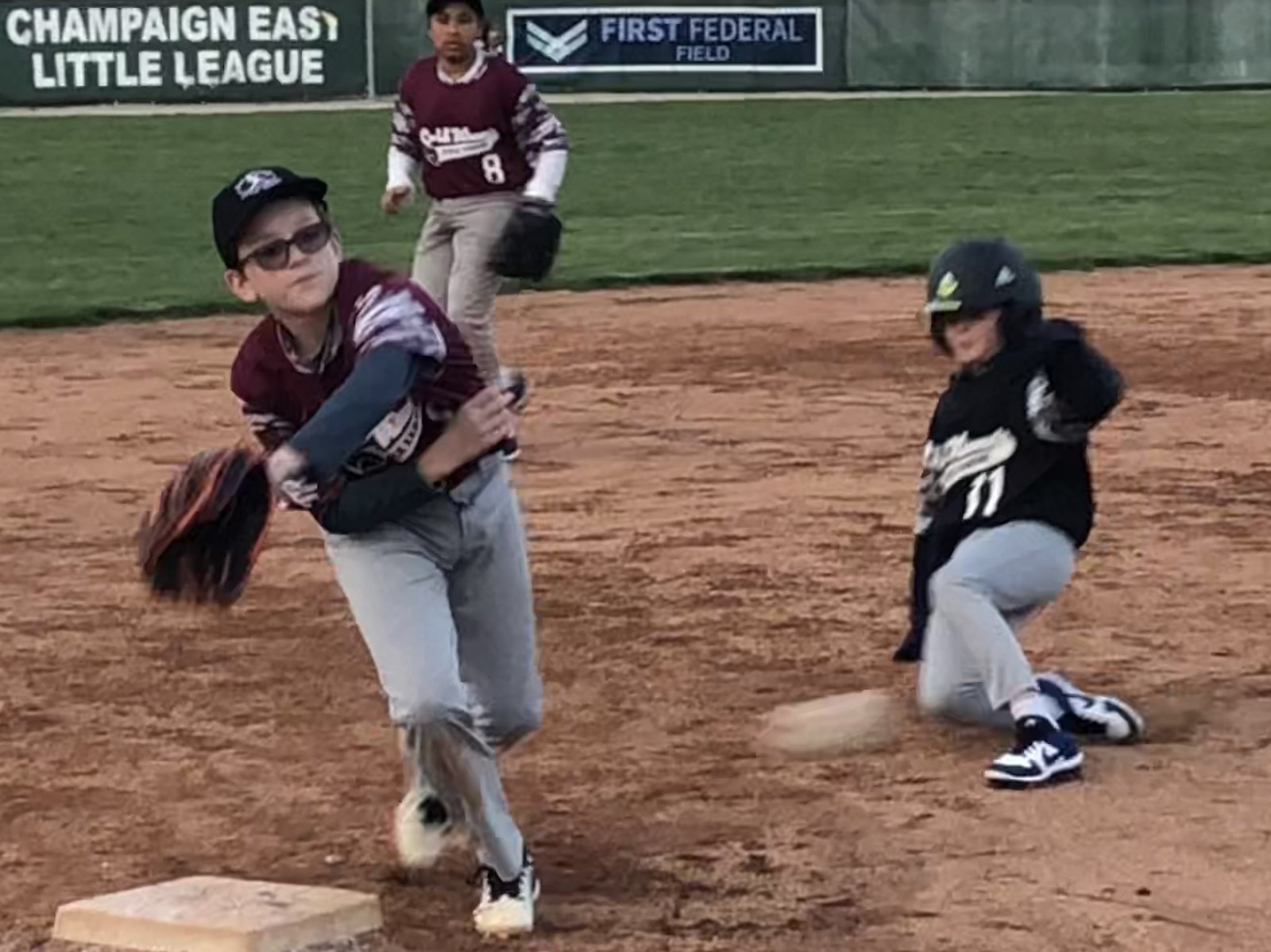The image captures a lively baseball game featuring three young players, likely between the ages of 8 and 12. At the center of the action, a child wearing a black long-sleeve jersey and long pants is seen sliding into the base, kicking up dirt as they do so. Positioned near the base, another child in a maroon long-sleeve jersey with sunglasses is about to catch the ball with their left hand, poised and focused. In the background, a third player in a maroon long-sleeve jersey and sporting a catcher's mitt watches intently. The setting includes a grassy field with green walls adorned by advertisements, one for "First Federal Field" and another for "Campaign East Little League," creating an authentic small-town baseball atmosphere.